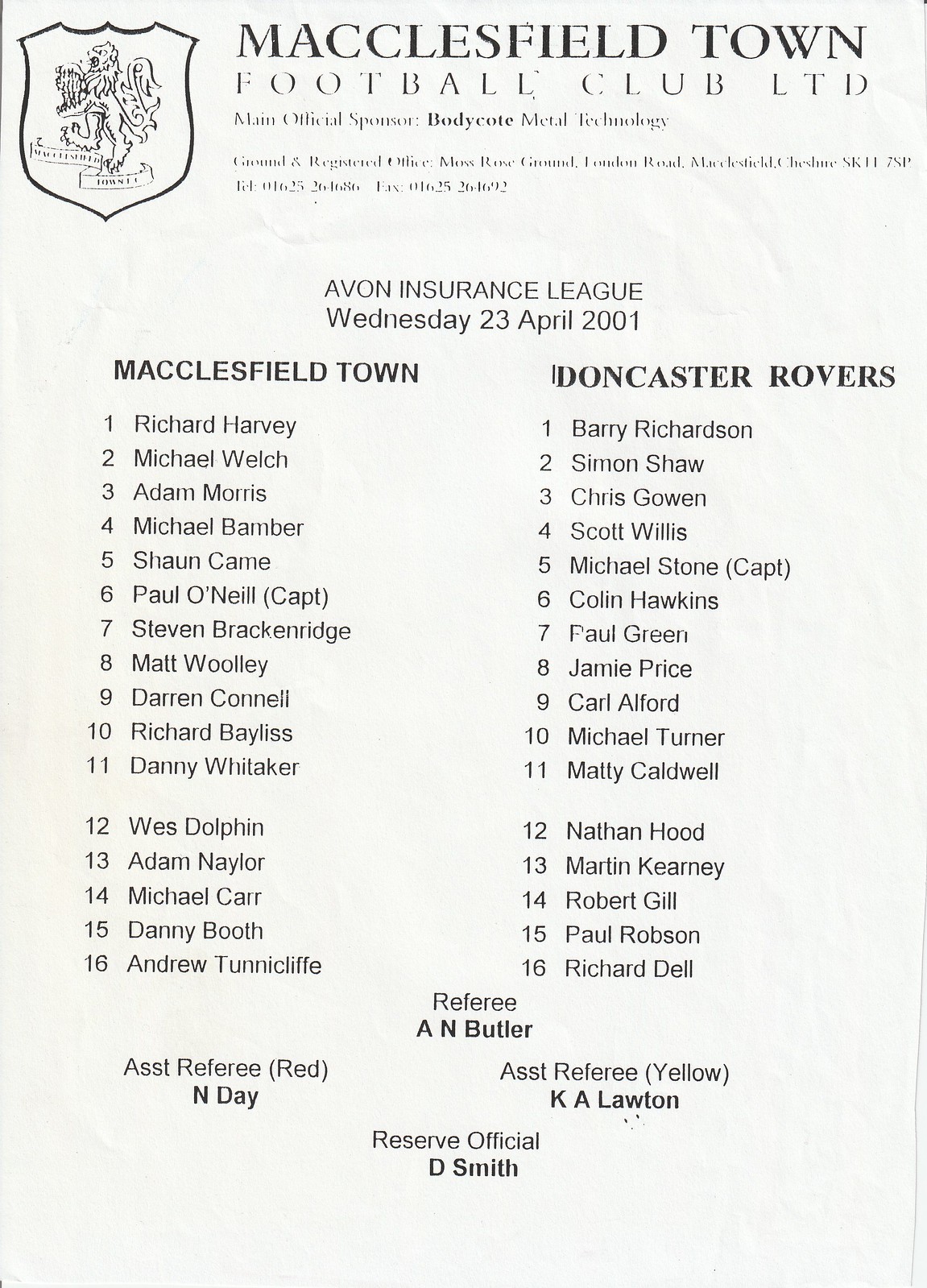This is a document from the Macclesfield Town Football Club Ltd., showcasing the match details for a game played on Wednesday, 23rd April 2001 as part of the Avon Insurance League. The upper left corner features a griffin crest. Printed at the top right under "Macclesfield Town Football Club, LTD" is the text "Main Official Sponsor Body Coat Metal Technology." Below, there is clear, black lettering on white paper, which appears slightly wrinkled, especially at the top.

The central part of the document, center justified about a third of the way down, highlights the title "Avon Insurance League, Wednesday 23rd April 2001." Moving down, the document lists the team members in two columns: the left column for Macclesfield Town and the right column for Doncaster Rovers, each listing the numbers 1 through 16 alongside the players' names.

At the bottom, the names of the match officials are displayed—centered and justified. The referee’s name is at the center, and directly beneath that, the names of the assistant referees, labeled "red" and "yellow," are listed. The name of the reserve official, D.E. Smith, appears beneath the assistant referees’ names.